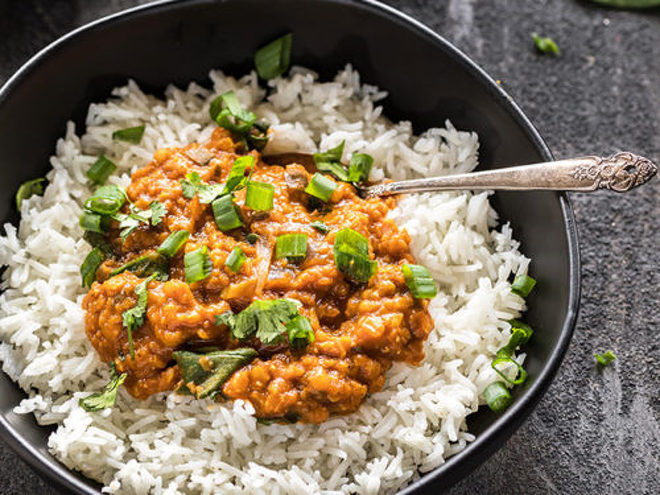The image depicts an aesthetically arranged bowl of food, prominently featuring short-grain white rice that is characteristic of sushi or other Japanese dishes. The rice, fluffy and pristine, is served in a simple, elegant black bowl that might be crafted from a stone-like material, potentially cobalt black in appearance. At the center of the rice sits a generous heaping portion of natto, a traditional Japanese dish made from fermented soybeans. The natto is garnished with finely chopped green onions, adding a fresh, vibrant touch to the dish. A silver spoon is delicately dipped into the center, untouched, suggesting the image was captured for aesthetic or promotional purposes. The bowl rests on a sleek, dark gray steel countertop, with the overall scene bathed in natural lighting that highlights the clarity and details of the meal.